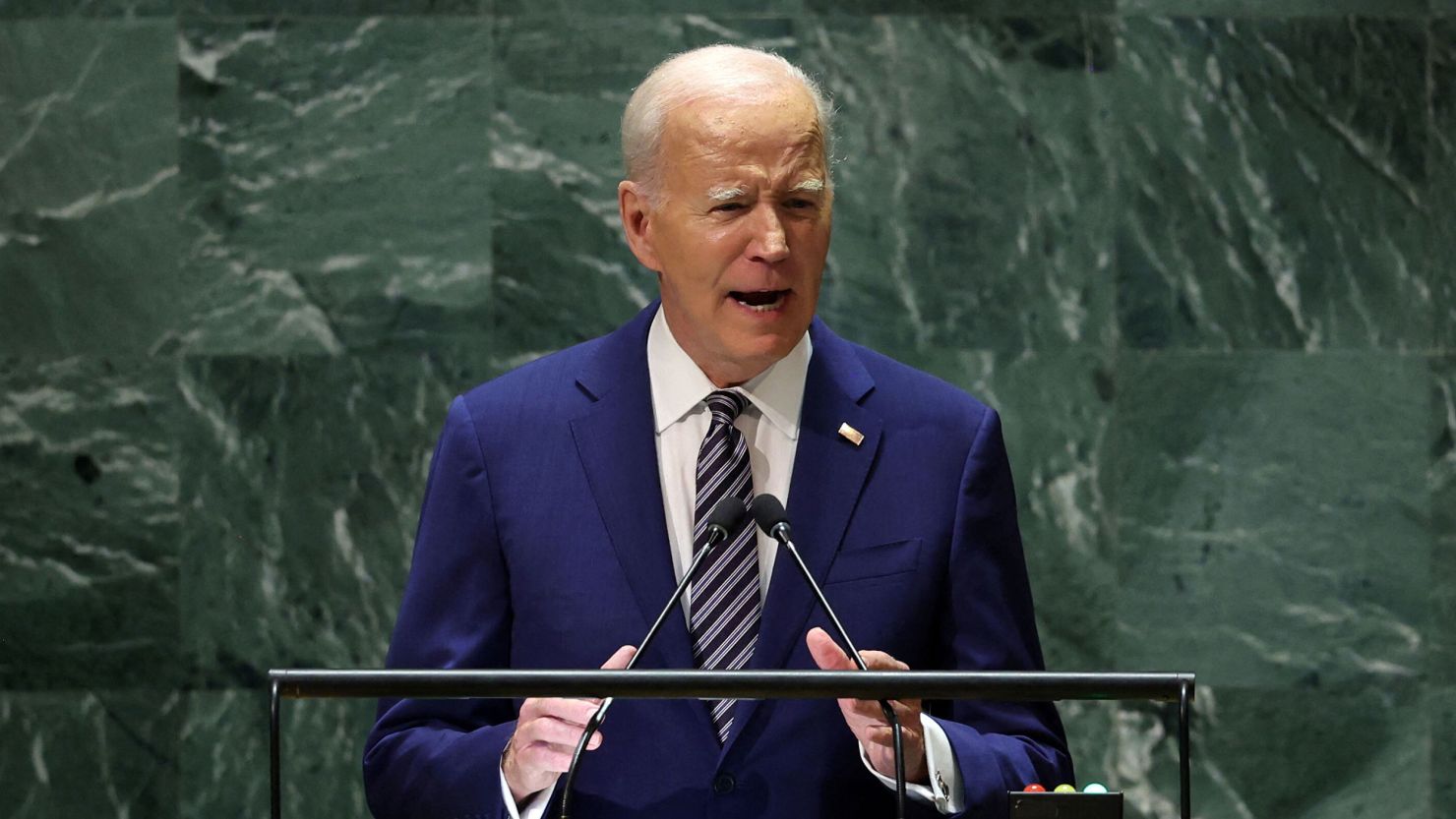This detailed photograph captures an elderly Joe Biden, the President of the United States, delivering a speech at a podium. He appears to be around 80 years old and is dressed in a navy blue suit complemented by a blue and white striped necktie. His attire is completed with a white undershirt. The scene is characterized by two small black microphones arranged in a triangle shape at the podium, aimed towards each other.

Joe Biden, showing signs of age with many visible wrinkles and balding, short white hair, also sports large white eyebrows reminiscent of caterpillars. His expression conveys a mixture of intensity and tiredness, with his mouth wide open and his forehead prominently wrinkled, suggesting a moment of passionate speech.

The backdrop consists of large green and gray marble tiles, adding a dignified ambiance to the setting. Additionally, a little rectangular box with three buttons—red, green, and white—is situated by his left arm, contributing to the intricate details of the scene. The overall impression is a vivid portrayal of a seasoned leader deeply engaged in his address.